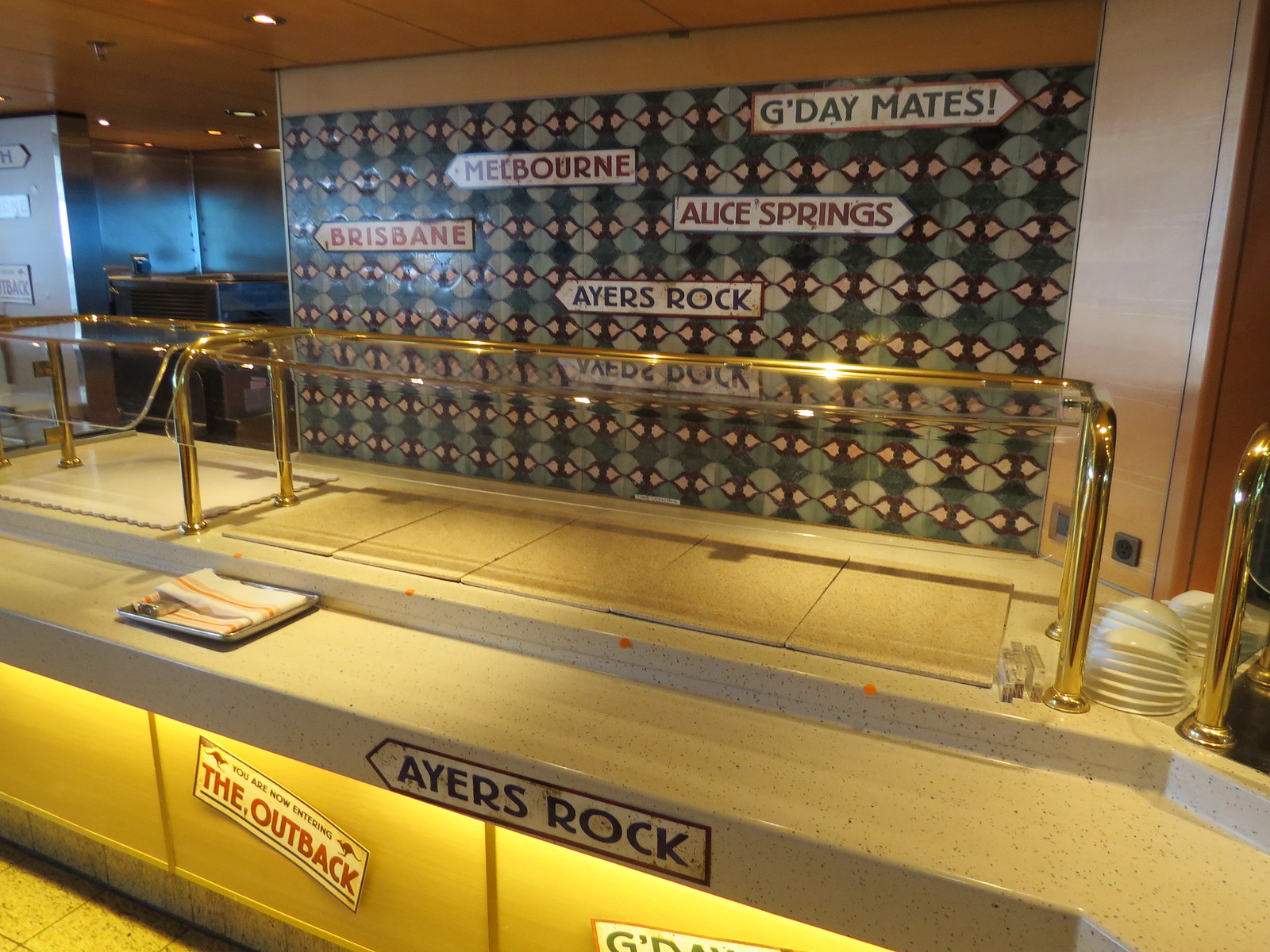The image depicts an indoor setting, likely a bakery or restaurant, centered around a buffet-style counter with a glass case designed to hold food, though it appears empty at the moment. Off to the far right, stacks of white bowls are neatly arranged. The surrounding environment is equipped with linoleum tile flooring, adding a practical touch to the decor. Dominating the back wall are multiple arrows pointing in various directions with place names such as "G'day Mates," "Melbourne," "Alice Springs," "Brisbane," "Ayers Rock," and "The Outback" inscribed on them, hinting at an Australian theme. The overall color palette includes shades of tan, yellow, red, white, gray, gold, green, brown, and maroon. The setting seems well-lit, suggesting it is daytime, and the layout implies a welcoming, yet orderly, dining atmosphere.